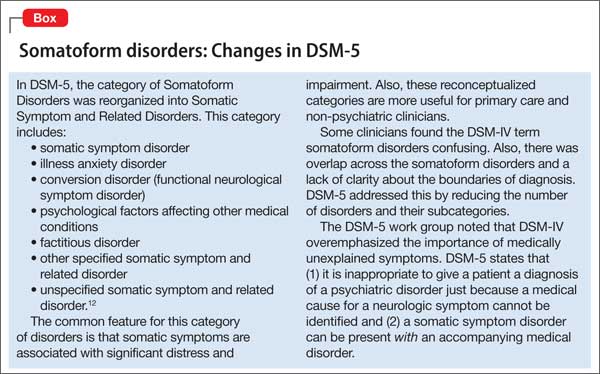This image is horizontally rectangular with a clean white background bordered by a fine black line. In the top section, a small red rectangle occupies the top left corner. The word "Box" is printed in white, with a capital 'B' followed by lowercase 'o-x'. Extending from the left side of this red box is a short horizontal line connected to a vertical line, forming an upside-down 'L' shape.

Below this, a bold headline in black font reads: "Somatiform Disorders: Changes in DSM-5." The headline emphasizes "DSM-5" in all capital letters, followed by a dash and the numeral "five."

The lower part of the image transitions into a light blue section, still framed by the thin white border on the bottom and sides. In this blue section, black text explains the reclassification of somatiform disorders in DSM-5. The text reads:

"In DSM-5, the category of somatiform disorders was reorganized into somatic symptom and related disorders. This category includes:
- Somatic symptom disorder
- Illness anxiety disorder
- Conversion disorder (functional neurological symptom disorder)
- Psychological factors affecting other medical conditions
- Factitious disorder
- Other specified somatic symptom and related disorder
- Unspecified somatic symptom and related disorder."

Beneath the bullet points, further information is provided in standard paragraph format:

"The common feature for this category of disorders is that somatic symptoms are associated with significant distress and impairment. Also, these reconceptualized categories are more useful for primary care and non-psychiatric clinicians. Some clinicians found the DSM-IV term 'somatiform disorders' confusing. Additionally, there was overlap across the somatiform disorders and a lack of clarity about the boundaries of diagnosis. DSM-5 addresses this by reducing the number of disorders and their subcategories. The DSM-5 workgroup noted that DSM-IV overemphasized the importance of medically unexplained symptoms. DSM-5 states that:
1. It is inappropriate to give a patient a diagnosis of a psychiatric disorder just because a medical cause for a neurologic symptom cannot be identified.
2. A somatic symptom disorder can be present with an accompanying medical disorder."

This detailed description of the image underscores the reorganization of somatiform disorders in DSM-5, offering clarity for both primary care and non-psychiatric clinicians.